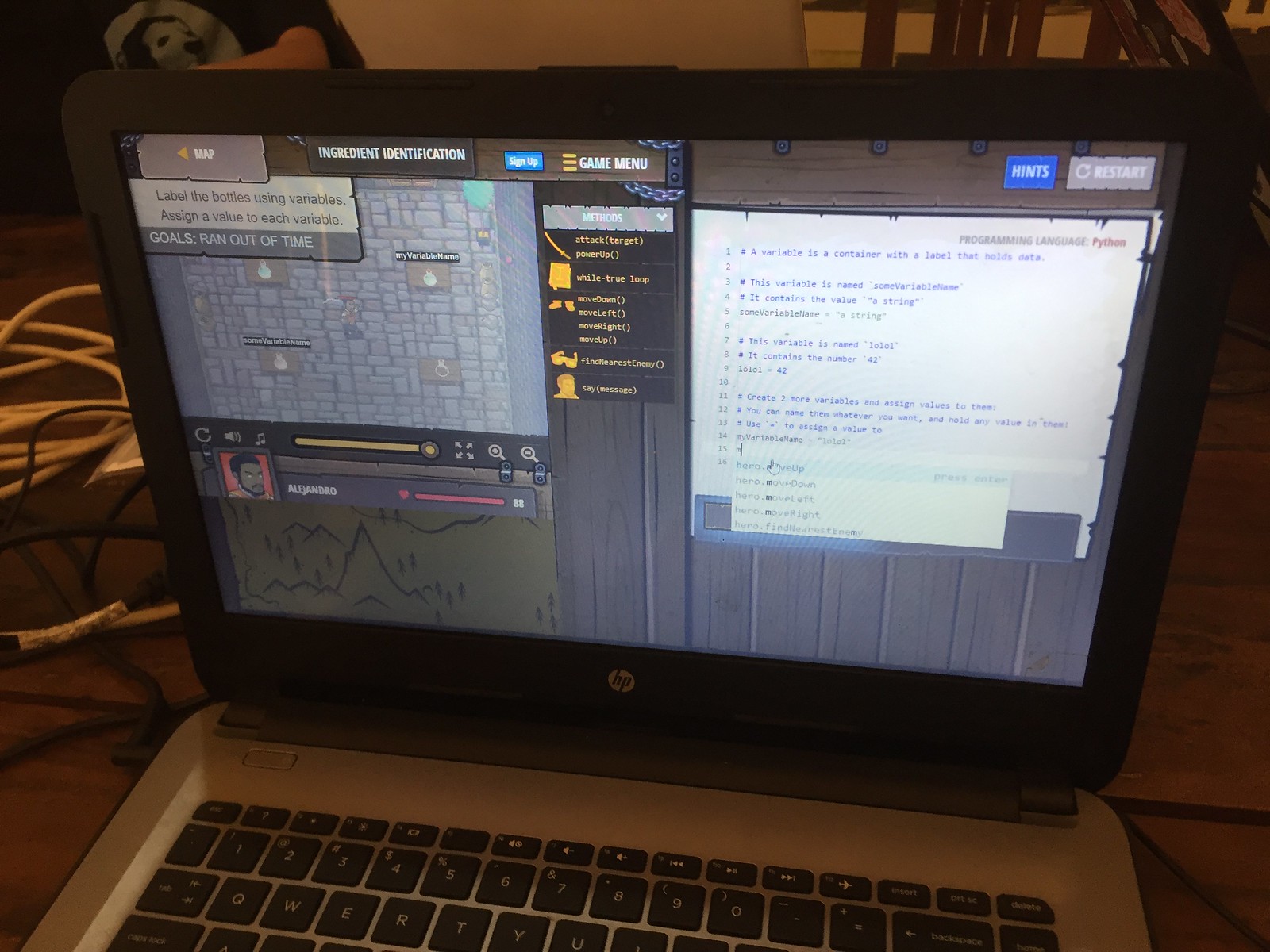The image depicts a complex computer screen filled with multiple overlays and windows, suggesting that it is from a video game. The top of the screen features several tabs labeled "Map," "Ingredient Identification," "Game Menu," "Sign Up," and "Goals." Text indicates that the player has "ran out of time" and includes instructions to "label the bottles using variables" and "assign a value to each variable."

Amidst the game interface, there are programming elements present, such as methods and a "while true" loop. A message can be seen, although the text is not entirely legible. This suggests the game is either designed to teach programming in an interactive, gamified manner or shows the development process of a game. Therefore, it is somewhat obscured whether the focus is on gameplay or on the backend development activities.